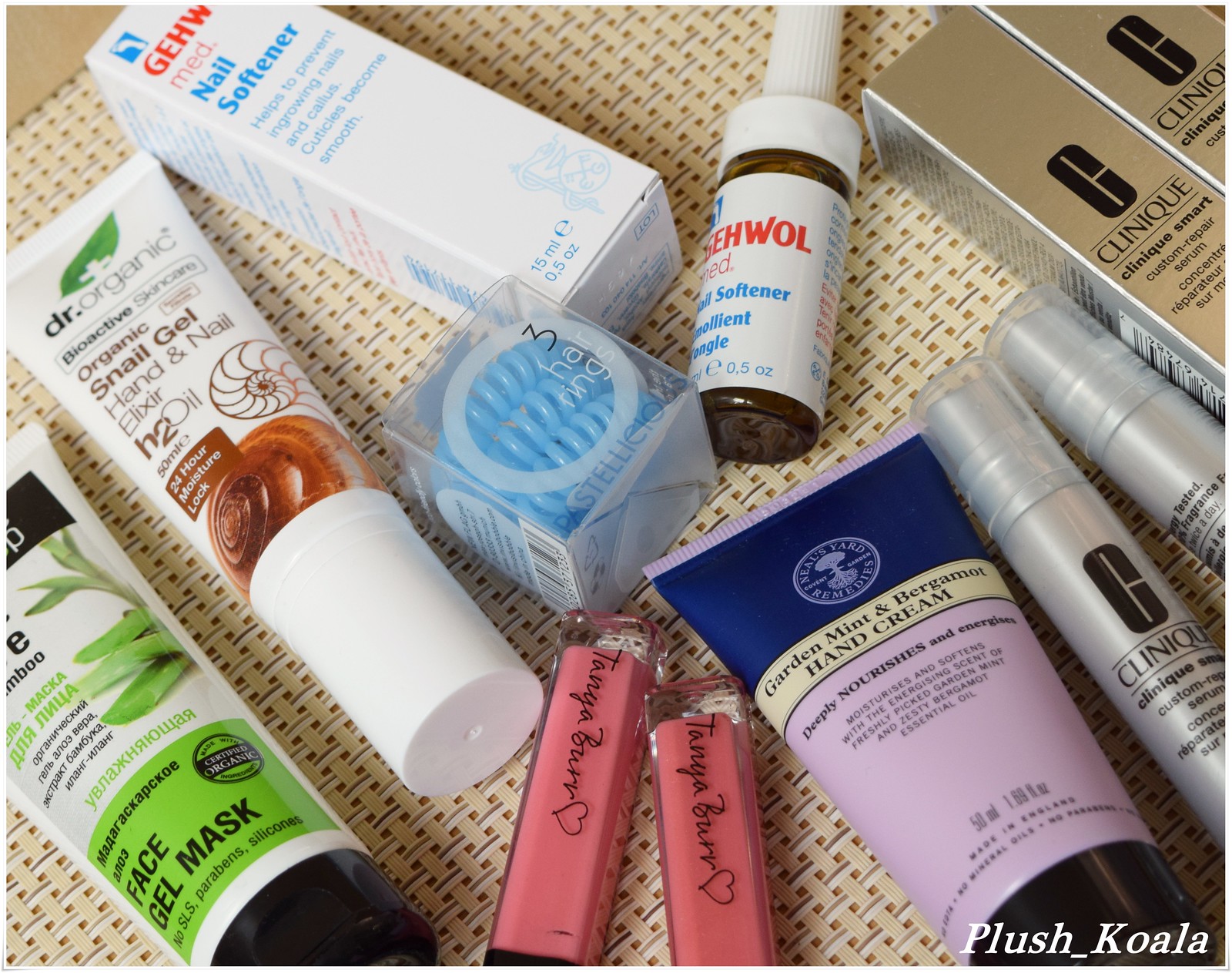The image features a collection of gels and creams arranged against a yellow background with small perforations and white and gray lines creating numerous tiny sections. In the bottom right corner, white lettering spells out "plush_cola."

In the foreground, there is a purple hand cream labeled "Garden Mint and Bergamot," which has a blue top and a black cap. Nearby are two Clinique custom eyeliners, each with a plastic cap. Accompanying them are two silver Clinique boxes with the iconic black letter "C" on them. The bottles inside the boxes are silver but less shiny than the packaging, each featuring a barcode on the side.

At the top left of the arrangement is a boxed product labeled "GEHWOL Med Nail Softener," designed to help prevent ingrown nails and calluses. The box has red and blue lettering on a white background, and the corresponding bottle—which has a white cap and dark gray body with white labeling—is positioned just to the right.

In the middle of the arrangement is a clear plastic box containing three bluish rings. To the left, you’ll find an Organics nail gel in a brown bottle labeled "Hand and Nail Elixir, H2O Oil," which features a white cap, brown swirls, and some white accents on the bottle itself, along with a Dr. Organic logo that includes a green leaf and a white cross.

Adjacent to this is a face gel mask with black lettering on a green background, complemented by a black cap. The white bottle displays an image of bamboo shoots.

At the bottom are two bottles of a product that appears to be labeled "Tangle Barn" or "Tanga Barn," each characterized by a red heart design. The liquid inside these bottles is pink, and they are topped with black caps.